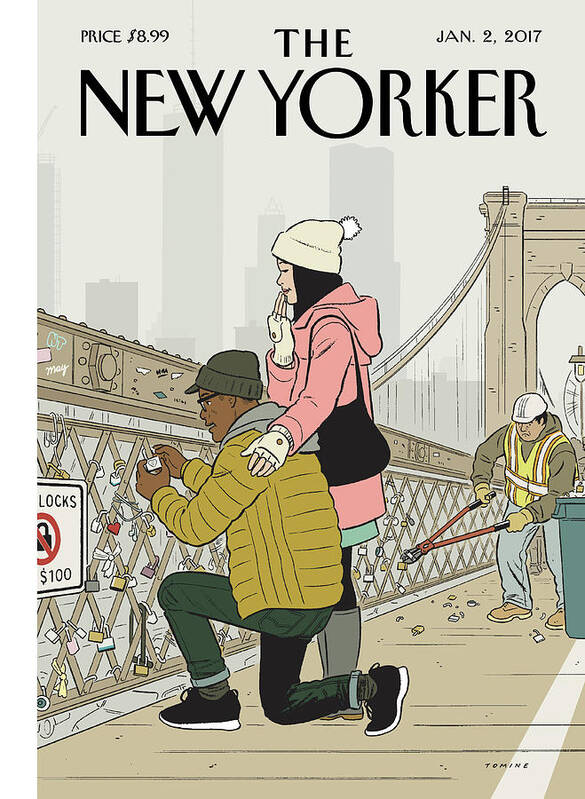This is an illustration on the cover of The New Yorker magazine, priced at $8.99, dated January 2, 2017. The cover prominently features The New Yorker's black logo at the top. The drawing showcases a suspension bridge in the background, likely inspired by iconic bridges like the Brooklyn Bridge. In the foreground, a black man and an Asian woman are kneeling down, the man securing a padlock with a heart on a fence attached to the bridge. The fence is cluttered with dozens of similar locks from other couples. To the left of the couple, a sign reads "No Locks," indicating a $100 fine for attaching locks. Further to the left, a sanitation worker equipped with a bolt cutter is actively removing the padlocks, with the removed locks falling to the ground and a trash can beside him for disposal.